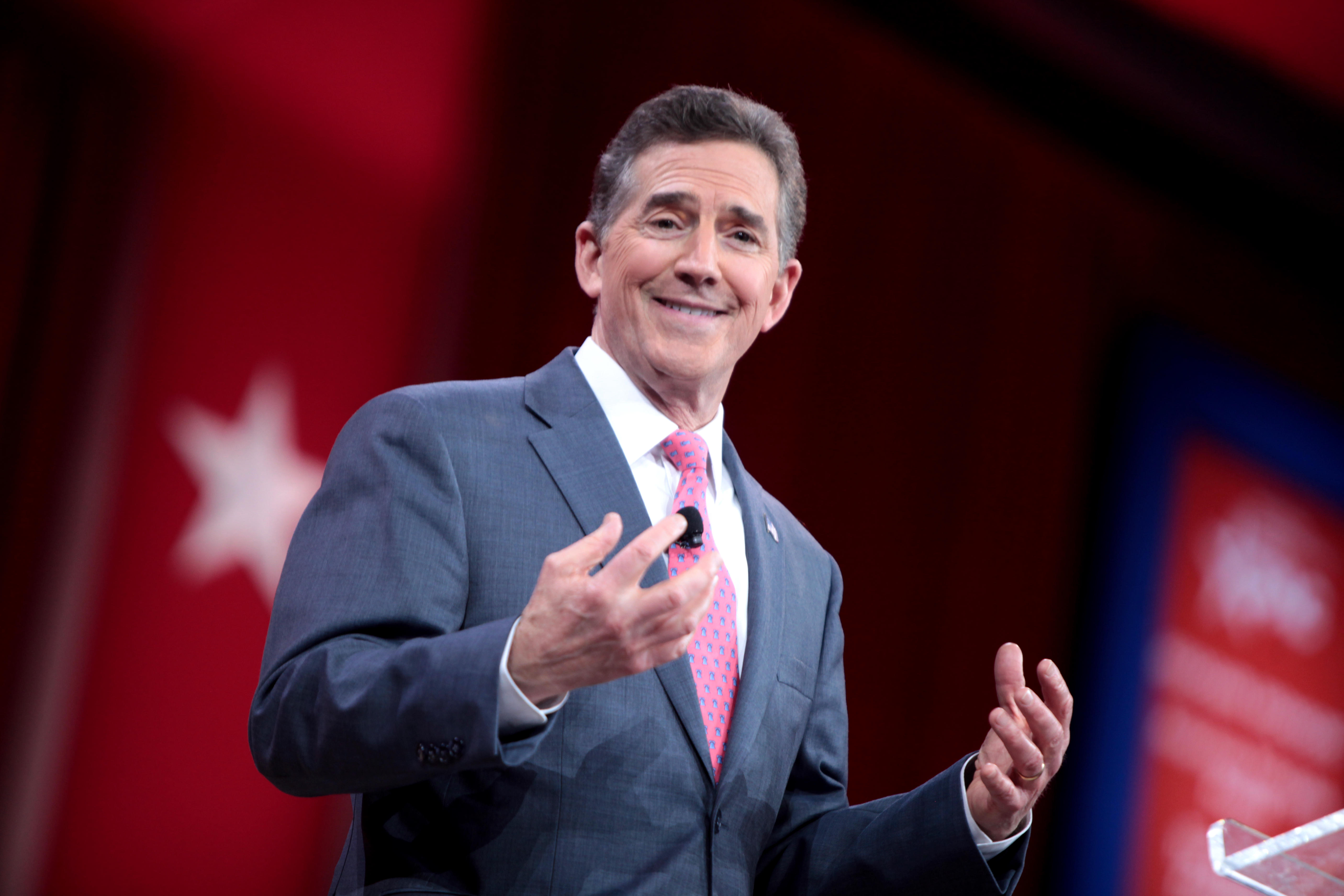The image depicts a man, possibly a politician in his 50s or 60s, standing on stage and engaging with the audience, who appears to be staring directly into the camera. He has short gray-brown hair and is dressed in a light gray jacket, a white dress shirt, and a pink or purple tie adorned with blue dots, with a heart-shaped or flag pin on the jacket’s lapel. The man is gesturing expressively with both hands in front of his chest, indicating he is in the midst of a speech. He also has a microphone clipped to his tie. Behind him, the background is out of focus but features red banners and curtains with white stars, suggestive of a campaign or patriotic event. A clear acrylic or glass podium is partially visible at the bottom right corner of the frame.